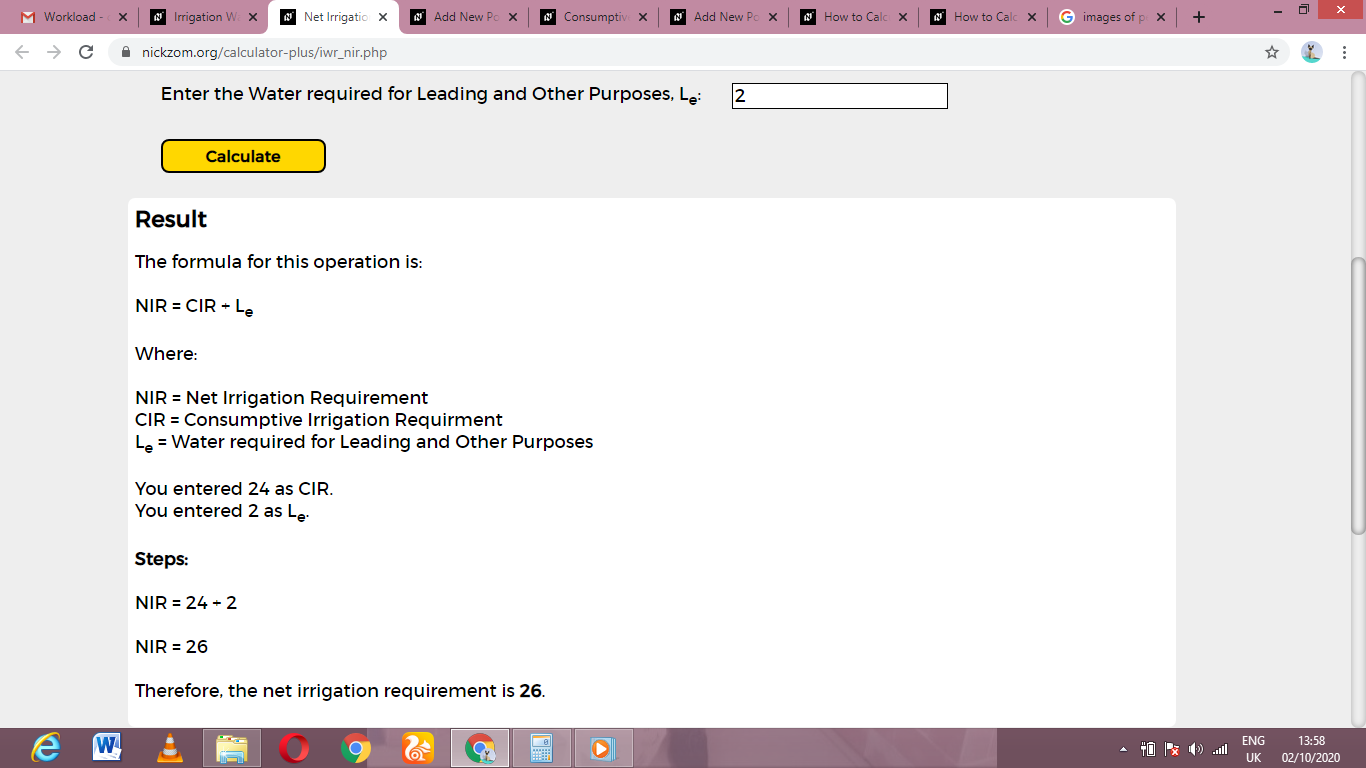A cluttered browser window showcases multiple tabs with a distinct pink theme on the top bar, indicating a personalized aesthetic. From left to right, the tabs read: "Workload" with a Gmail icon, "Irrigation W" (cut off), "Net Irrigation" (cut off), "Add New PO," "Consumption" (cut off), another "Add New PO," followed by two instances of "How to CALC" (both cut off). The next tab is a Google image search titled "Images of P" (cut off).

In the URL bar, the user has typed "nickzom.org/calculator-plus/IWR_NIR.php." The main screen, set against a light gray background, features a black header that begins with "Enter the water required for leading and other purposes LE" (cut off). On the right, there's a white search field containing the number two. Below this, to the left, is a yellow rectangular button with a black rounded border reading "Calculate" in bold.

In the top left corner of the page, a white square area titled "Result" in bold black letters contains a detailed formula explanation for the necessary operation, starting with "The formula for this operation is:" followed by a methodical description of the steps involved in solving the equation.